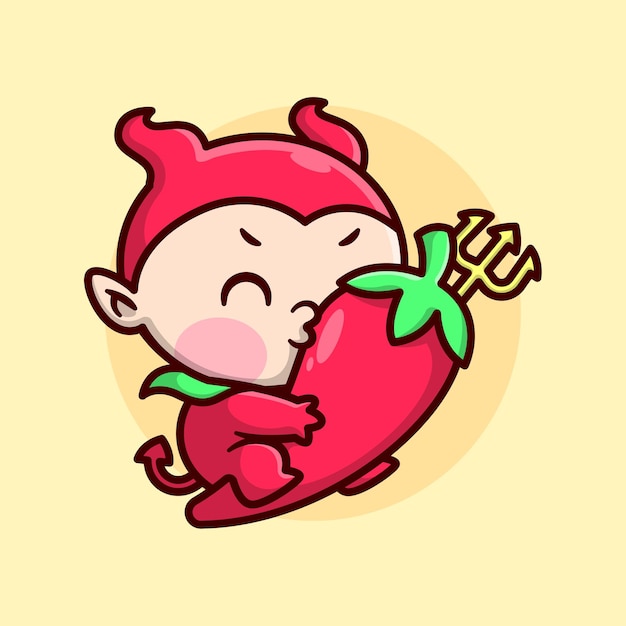This whimsical, computer-illustrated image features a chubby, child-like devil figure, adorned with a red hat and red horns, pointy ears, and bright pink circular cheeks, adding to its cute, "kawaii" appearance. The devil wears a green collar or cape around his neck, complementing his red outfit and forked tail, which points upwards. With closed eyes and a joyful expression, the devil is seen hugging and kissing a large red chili pepper with a green leafy top, the stem of which points towards the upper right-hand corner. The gold pitchfork he holds is partially visible, protruding from behind the pepper. The illustration is set against a darker yellow circle, centered on a lighter yellow background, enhancing its playful and enchanting aesthetic.